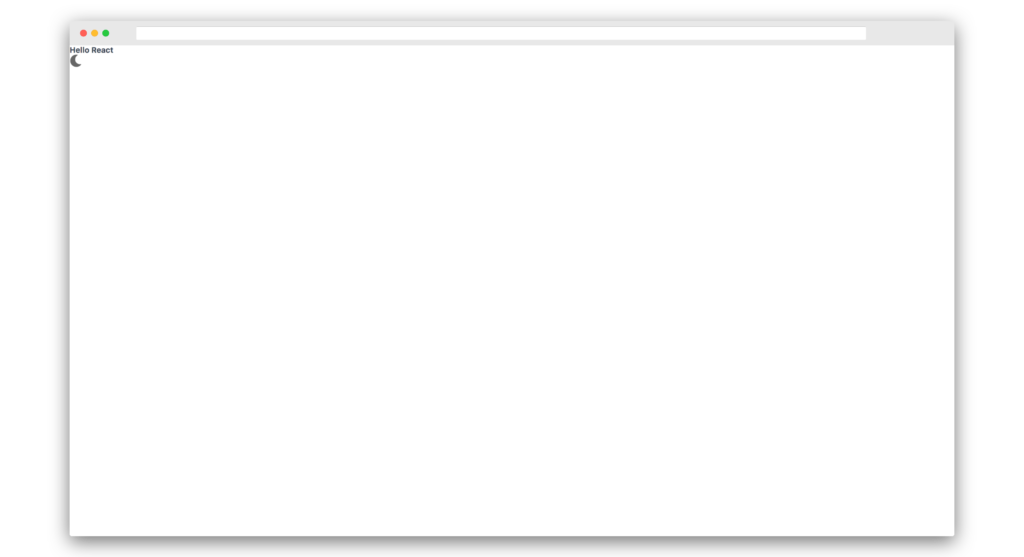The image is a screenshot of a blank interface. At the top left corner, there are three familiar Apple circles: a red circle, a yellow circle, and a green circle, representing the window control buttons. Below these circles, there is a white rectangular search bar set against a gray background. Centered beneath the search bar is the text "Hello React," with "Hello" capitalized as 'H' and in lowercase for 'e-l-l-o,' and "React" written with a capital 'R' followed by lowercase 'e-a-c-t.' Directly underneath this text is a small, darkish gray moon icon. The rest of the interface features a white blank space without any additional text, images, or elements. Surrounding the entire content area is a subtle halo shadow effect in a grayish tone, adding some visual depth to the otherwise minimalistic design.